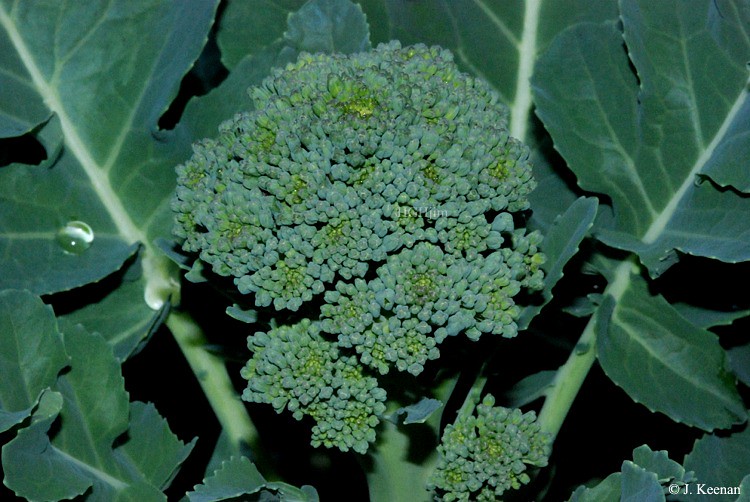This extreme close-up color photograph captures a broccoli floret nestled amidst broad green leaves. The floret is primarily a dusty green, composed of numerous tiny green buds, some of which have opened into small green leaves, adding texture and depth. Positioned to the left of the floret is a large leaf with a prominent white central vein, on which two drops of water gleam, reminiscent of how water beads on a waxed car. The plant's central stem, a light green in hue, extends downward and out of the frame. Surrounding the floret are several large, slightly out-of-focus leaves, contributing to the sense of depth. The background leaves and some smaller jagged-edged leaves at the image's corners create a rich, layered effect. There is also a copyright notice in white text at the bottom right corner, reading "J. Keenan." This detailed composition highlights the intricate structure and natural elegance of the broccoli within its leafy surroundings.